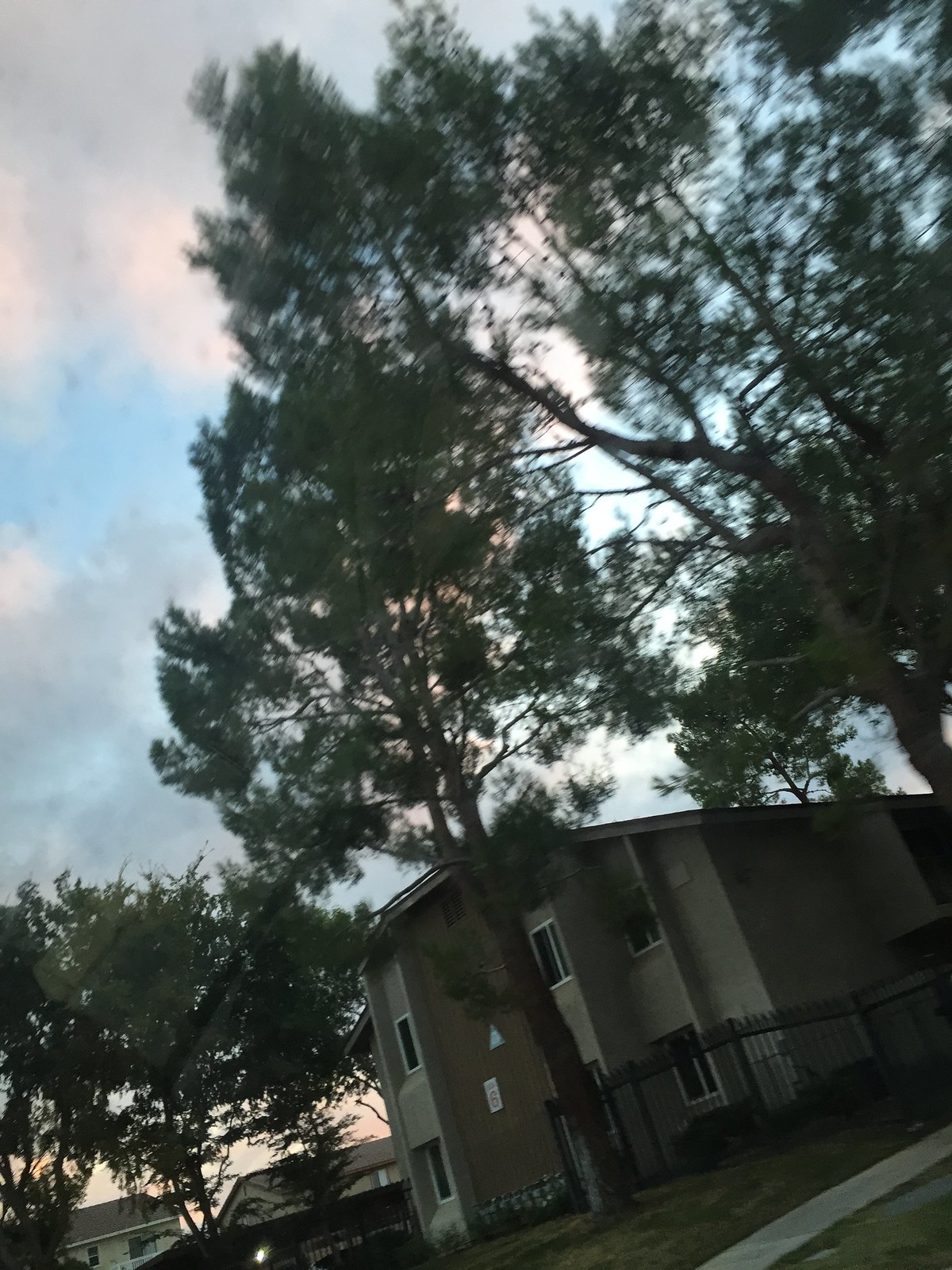The image prominently features an apartment building, specifically the narrower side of the structure which extends deeper into the scene. A red sign displaying the number six is visible, with an indistinct word above it. Adjacent to this is a triangular sign bearing a light blue interior and a white symbol. At the base of the building, several natural gas meters are present. Above these meters, there's a medium brown area that might represent a façade or a decorative element. The windows are framed by light gray surroundings, likely influenced by the lighting conditions.

The building has a sloped roof and is flanked by greenery, including shaded trees and a lawn that is partially brown and sparse in places. A black fence supported by vertical poles runs along the sides of the building. In the foreground, a cement sidewalk is visible.

To the lower left of the image, several additional structures appear. One has pale yellow sides with a brown roof, while another is tan-colored with a similar brown roof. The sky showcases a diverse palette of colors, including shades of light blue, blue, light pink, gray, white, and black, indicative of a transitional time of day, possibly dusk or dawn.